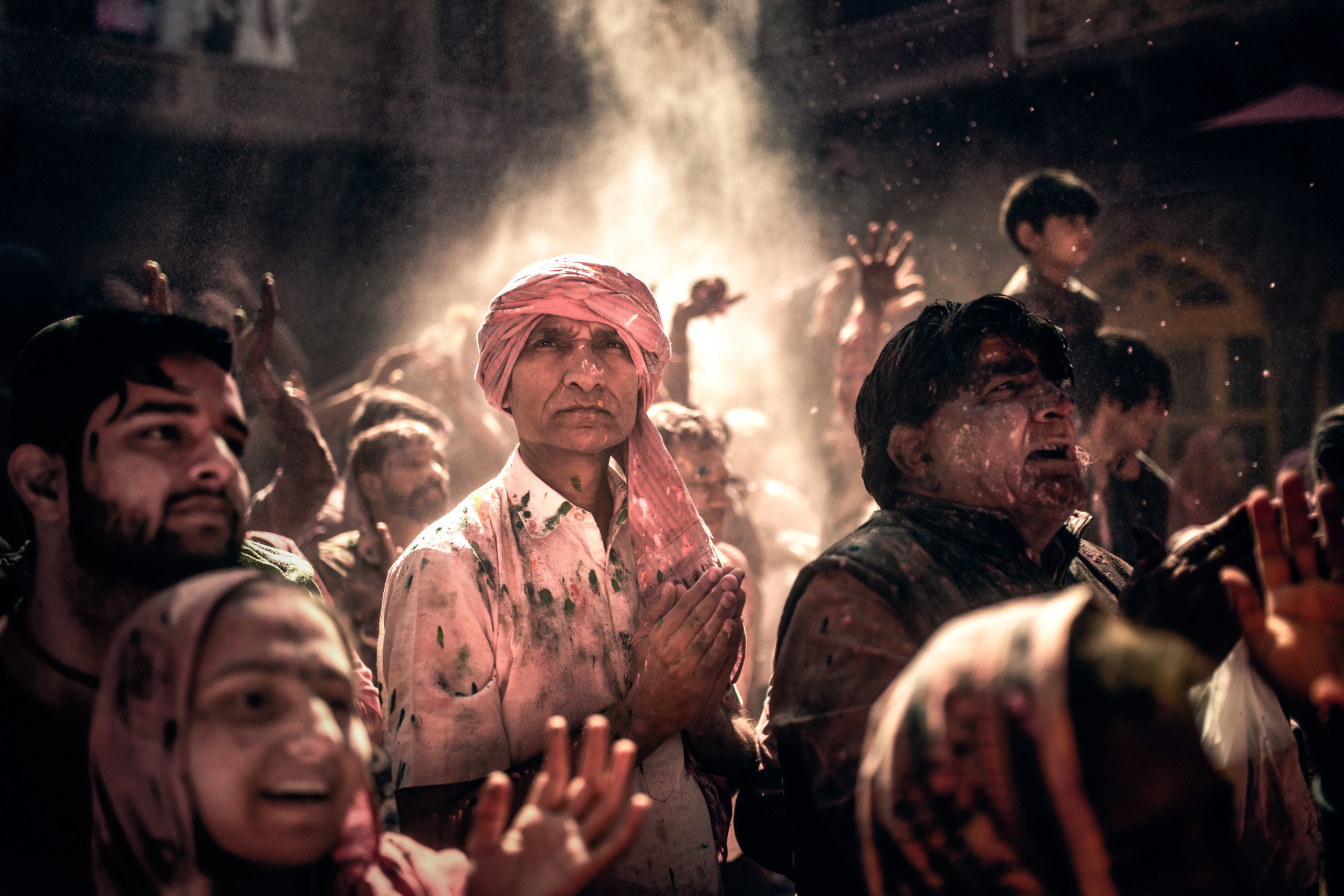The photograph captures a vibrant outdoor scene during the daytime, lit naturally by sunlight. The main focus is a man in the center, prominently wearing a red turban and a white shirt smeared with colored powders, suggesting he is participating in the Indian festival of colors, known as Holi. His hands are positioned together as if in prayer, though he could also be caught mid-clap. Surrounding him is a diverse crowd of people, including men, women, and children, all visibly excited and celebrating, some with arms raised and smiles on their faces. The people on the sides are slightly out of focus but contribute to the lively atmosphere. The upper part of the image is darker, with white or gray smoke or mist diffusing from the top, adding to the festive ambiance. The background lacks distinct features but is framed by dark walls with yellow windows, enhancing the scene’s focus on the celebrants. Notable details include a man on the left with a star on his head, a woman on the front left in a red and black cloak, and various individuals dressed in dark clothing, including a child on someone’s shoulders in the back right. Overall, the image captures a spirited moment of communal joy and cultural tradition.